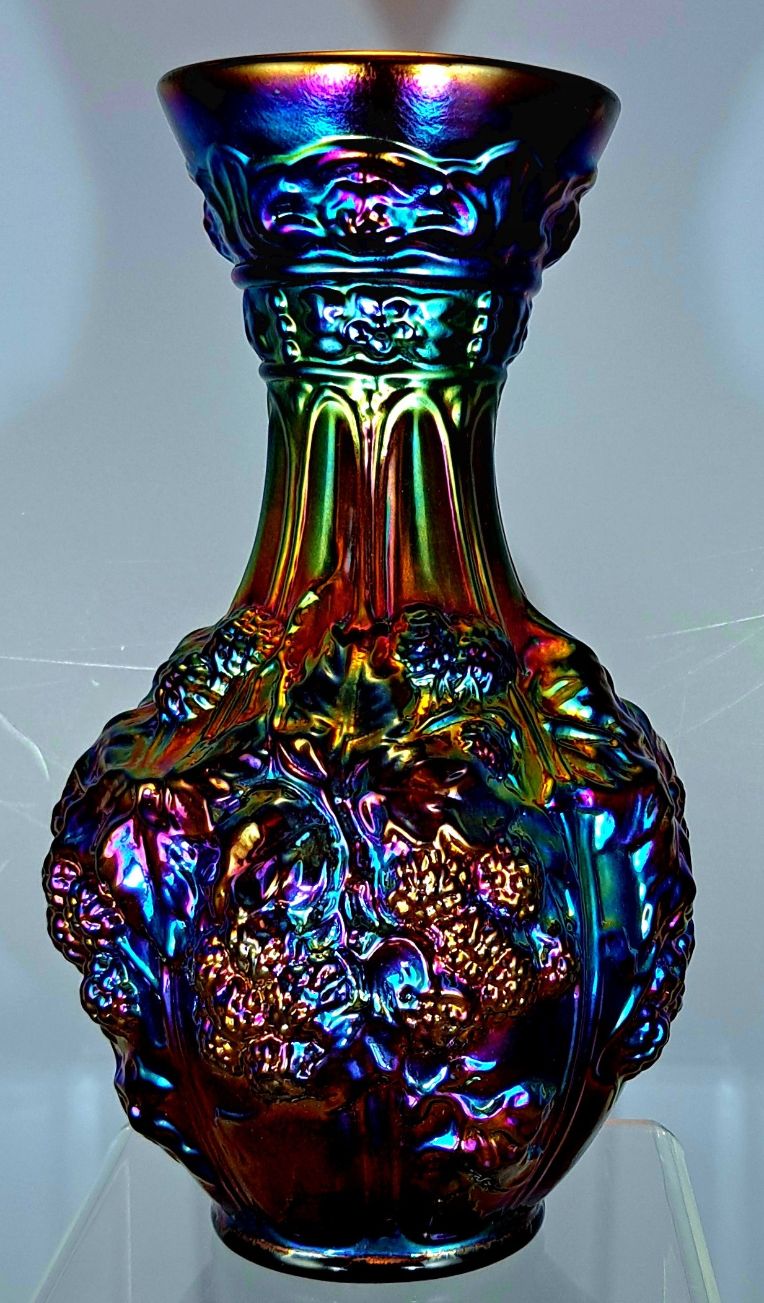The image features an exquisite vase made of dark blue carnival glass, renowned for its iridescent sheen that shimmers with metallic hues of gold, purple, green, violet, red, and blue. The vase showcases a detailed grape motif, seemingly molded into its design, evoking a sense of artistry and craftsmanship. It possesses a distinctive shape, with a wider mouth that elegantly narrows into a neck before expanding into a round body set upon a pedestal base. This intricate piece rests on what appears to be a translucent, see-through table or stand, which adds to the ethereal quality of the display. The background is a light blue or possibly grayish hue, which further accentuates the shadows and reflections of the multicolored vase, creating a stunning visual ensemble.